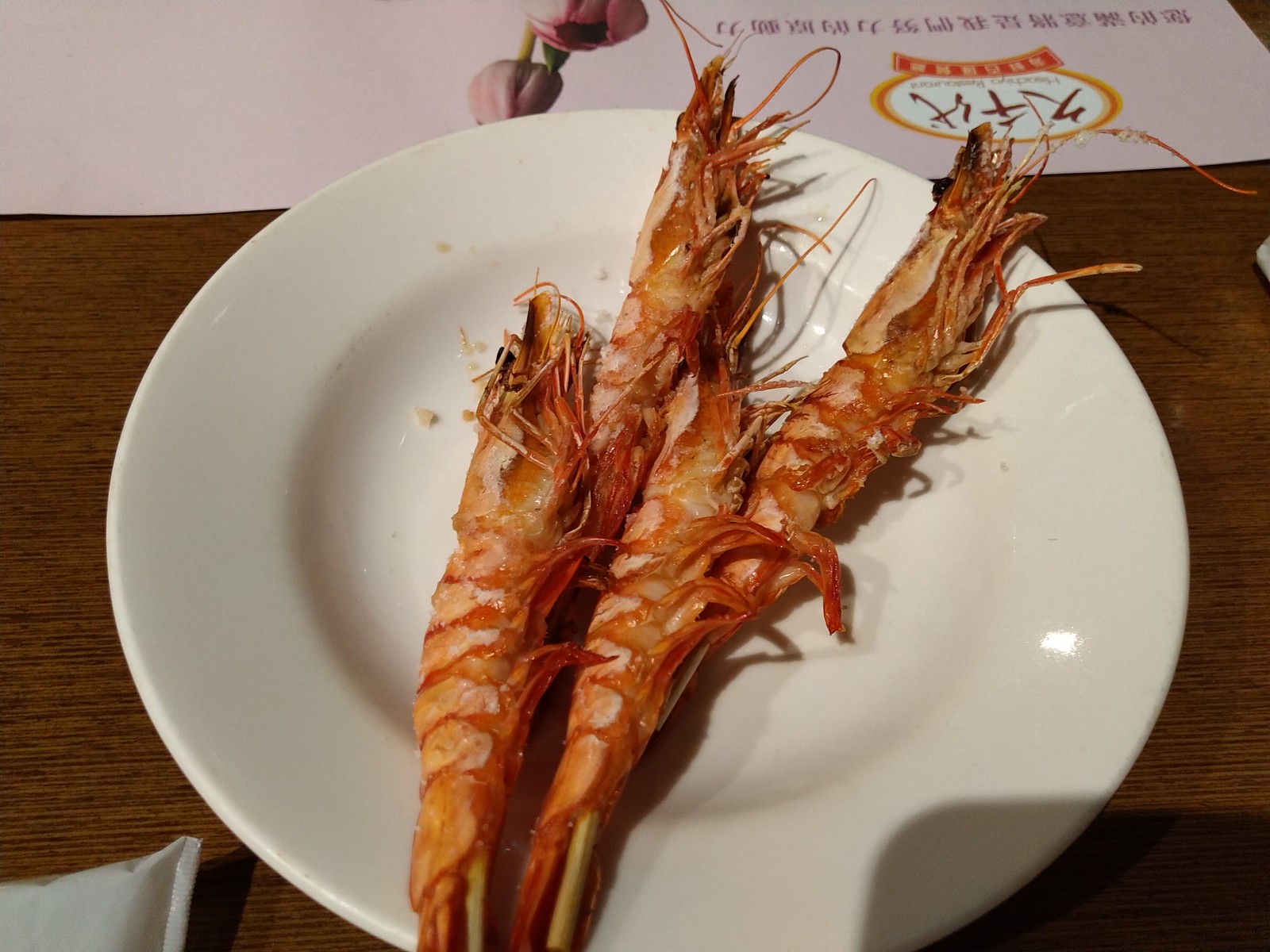This is a detailed photograph likely taken in a restaurant, showcasing a white plate with a wide brim, resembling a semi-bowl dish, placed on a brown wooden table with horizontal grain. The plate contains four large, whole prawns, skewered with sticks visible at their ends. The prawns appear to be either grilled or deep-fried, with all legs and heads still attached. Beneath the plate is an ivory-colored surface. In the background, there is an upside-down menu on the table featuring a pink background with Asian writing and a flower image. Additionally, a pink flower decoration is visible in the center of the table, adding to the elegant dining presentation.